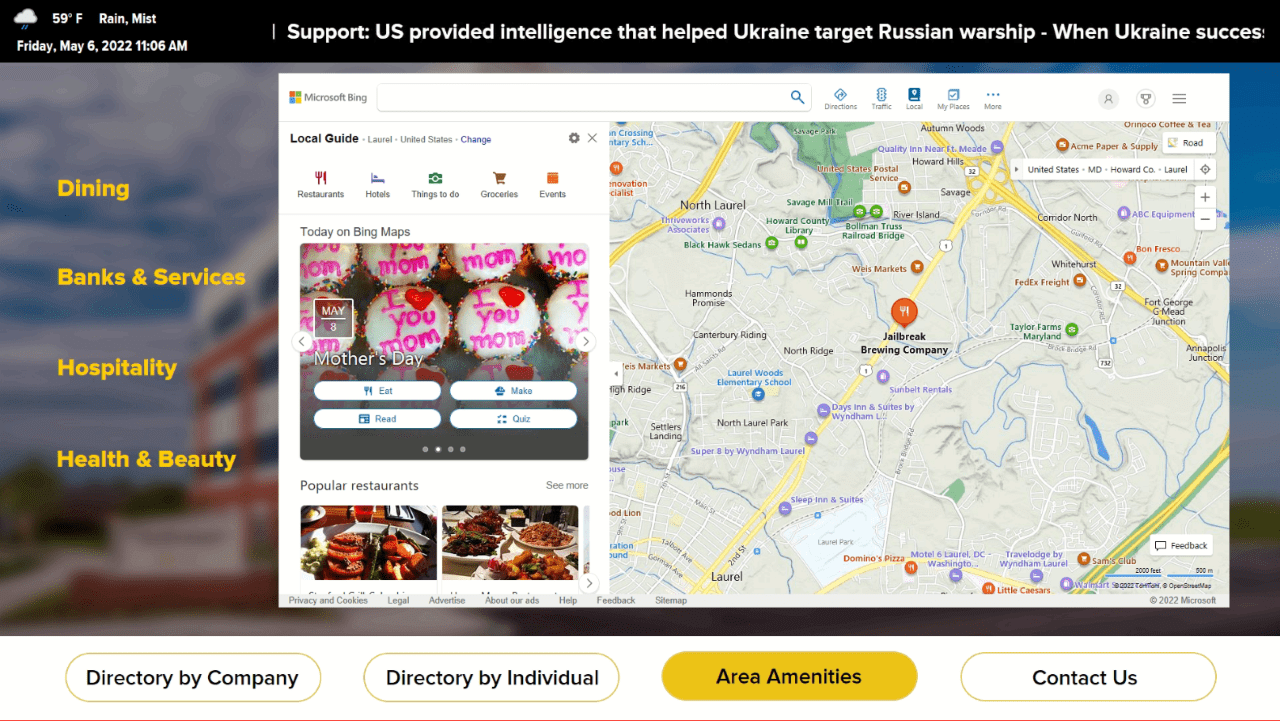Here's a cleaned-up and detailed caption for the image:

---

In the upper-left corner of the image, there's a weather indicator displaying "59°F," with rain and mist icons. Below this, a black strip stretches across the top, shown at "Friday, May 6, 2022, 11:06 a.m." The strip also contains a news headline: "Support provided intelligence that helps Ukraine target Russian warship," with a continuing phrase about Ukraine's success. 

On the left side of the image, four categories are listed in a column: "Dining," "Banks and Services," "Hospitality," and "Health and Beauty." 

The center of the image features a map, although the specific location is unclear. At the top of the map interface, various options are displayed: "Local Guide," "Laurel, United States," with options to change between "Restaurants," "Hotels," "Things to Do," "Groceries," and "Events." There are also icons for "Settings" and "Close." Additionally, "Today on Bing Maps" is visible, and "Microsoft Bing" is written across the top, accompanied by a search bar.

On the right side of the image, there's a photograph of cupcakes decorated with white frosting and pink icing, spelling out "I ♥️ you, Mom," tailored for Mother's Day. Below this, it prompts users with options like "Eat," "Read," "Make," and "Quiz." 

Further down, a section labeled "Popular Restaurants" is shown, featuring two photographs, and an option to "See More."